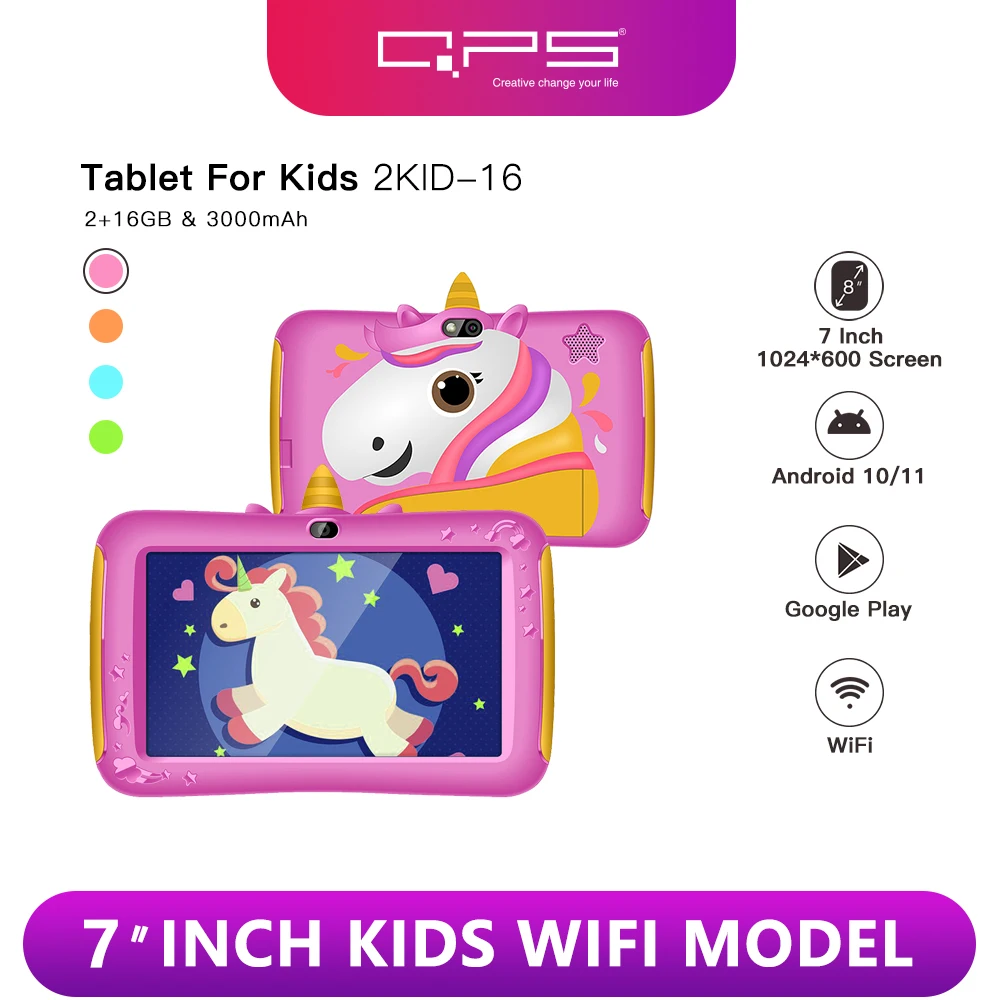The advertisement features a vibrant, color-rich design promoting a 7-inch kids' Wi-Fi tablet, detailed for a captivating visual appeal. The device, encased in a thick pink border adorned with shiny stars, showcases a whimsical unicorn theme. The front display includes a unicorn image on the screen, surrounded by an ombre pink to purple label at the top, which prominently reads "CPS" in white letters, alongside the slogan “Creative, change your life.” Beneath this, in black text, the tablet specifications are listed: “Tablet for kids, 2KID-16, 2 plus 16 gigabyte, and 3000 mAh.” Additional icons indicate color choices—pink (circled in black to indicate selection), orange, turquoise, and green.

The tablet's back is displayed above the front, highlighting a white unicorn with pink hair, a star-shaped speaker, and a camera, with the unicorn's horn centrally positioned. Details of the back's design include a large animated unicorn surrounded by emerald green stars and hearts. On the right-hand side of the ad, further information is listed: a 7-inch, 1024x600 screen, Android 10/11 compatibility, Google Play access, and Wi-Fi connectivity. A purple banner at the bottom emphasizes the model as the “7-Inch Kids Wi-Fi Model.” The entire presentation is animated with a playful, child-friendly aesthetic, ensuring it captures the imagination and interest of its young audience.